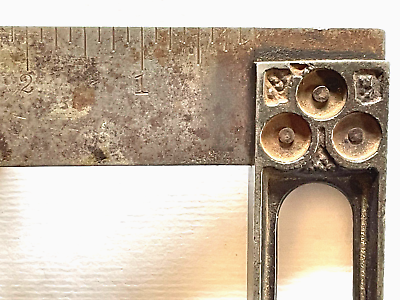The sepia-toned image captures a close-up of a vintage, rusted metal ruler, positioned horizontally from left to right, revealing markings up to about two and a quarter inches. The aged ruler, which once might have been silver, now displays a spectrum of tans, rusts, and whites, with noticeable speckles and rust marks indicating its antiquity. Resting against the right side of the ruler is a small, roughly half-inch wide rectangular metal object extending longer vertically than horizontally. This object features three circular indentations and arcs down on either side, suggesting it might be an old hardware component or antique tool. The background displays a two-toned wall with the upper part appearing brassy with vertical lines and the bottom lighter, possibly illuminated by sunlight. The image lacks any textual elements, focusing solely on the interplay of aged metal textures and the warm, nostalgic color palette.